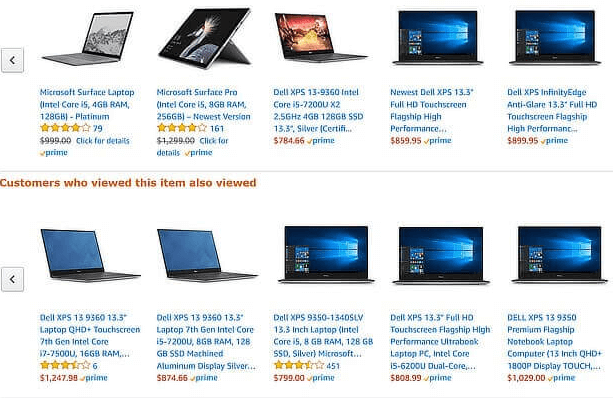The image depicts an Amazon shopping interface where a user is browsing laptops. There is a row of laptop options, navigable via an arrow to explore more selections. The highlighted laptops include a Microsoft Surface Laptop featuring an Intel Core processor, 40 GB of RAM, 79 reviews, and a 4-star rating. Another option is a Microsoft Surface Pro with an Intel Core processor, 8 GB of RAM, 161 reviews, and a 4-star rating. Additionally, there is a Dell XPS 13.9 360 with an Intel Core i5 processor, which currently has no reviews or stars.

Further down, items such as the latest Dell XPS 13.3 Full HD touchscreen model and the Dell XPS Infinity Edge Anti-Glare 13.3 Full HD touchscreen model are listed. At the bottom section, there's a "Customers who viewed this item also viewed" recommendation list. This includes a Dell XPS 13 9360 with a 13.3-inch screen, a Dell XPS 13 Laptop with a 7th generation Intel Core processor, and a Dell XPS 9350 with a 13.3-inch screen.